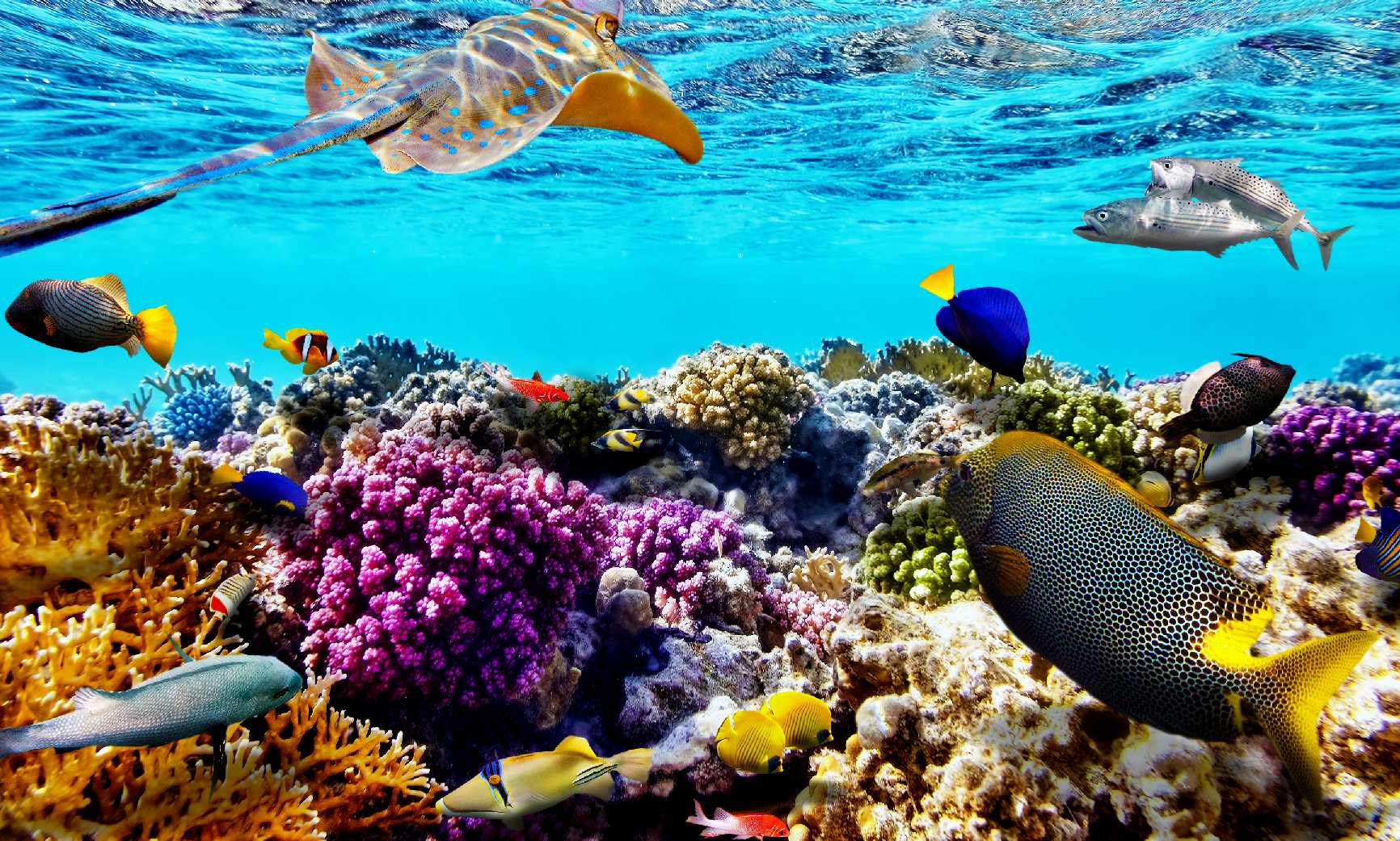This vibrant underwater photograph captures the deep blue sea in all its glory. The scene features a rich, clear blue ocean teeming with life, offering a prime spot for scuba diving. At the heart of the image, a variety of colorful fish—including cod, blue fish, yellow fish, and possibly an angelfish with a blue body and bright yellow tail—swim peacefully amid the coral reefs. The coral itself is a stunning array of oranges, bright pinks, grays, and tans. Near the seabed, smaller orange and white fish, perhaps clownfish, add to the diversity. There's even a glimpse of a stingray characterized by its brown and tan body adorned with blue dots. Purple and light blue hues under the sea reflect beautifully, while the surface waves create a serene backdrop. This captivating snapshot of oceanic life reveals an array of species like blue fish, yellow fish, fish with black spots, and small clownfish all coexisting in a tranquil underwater paradise.